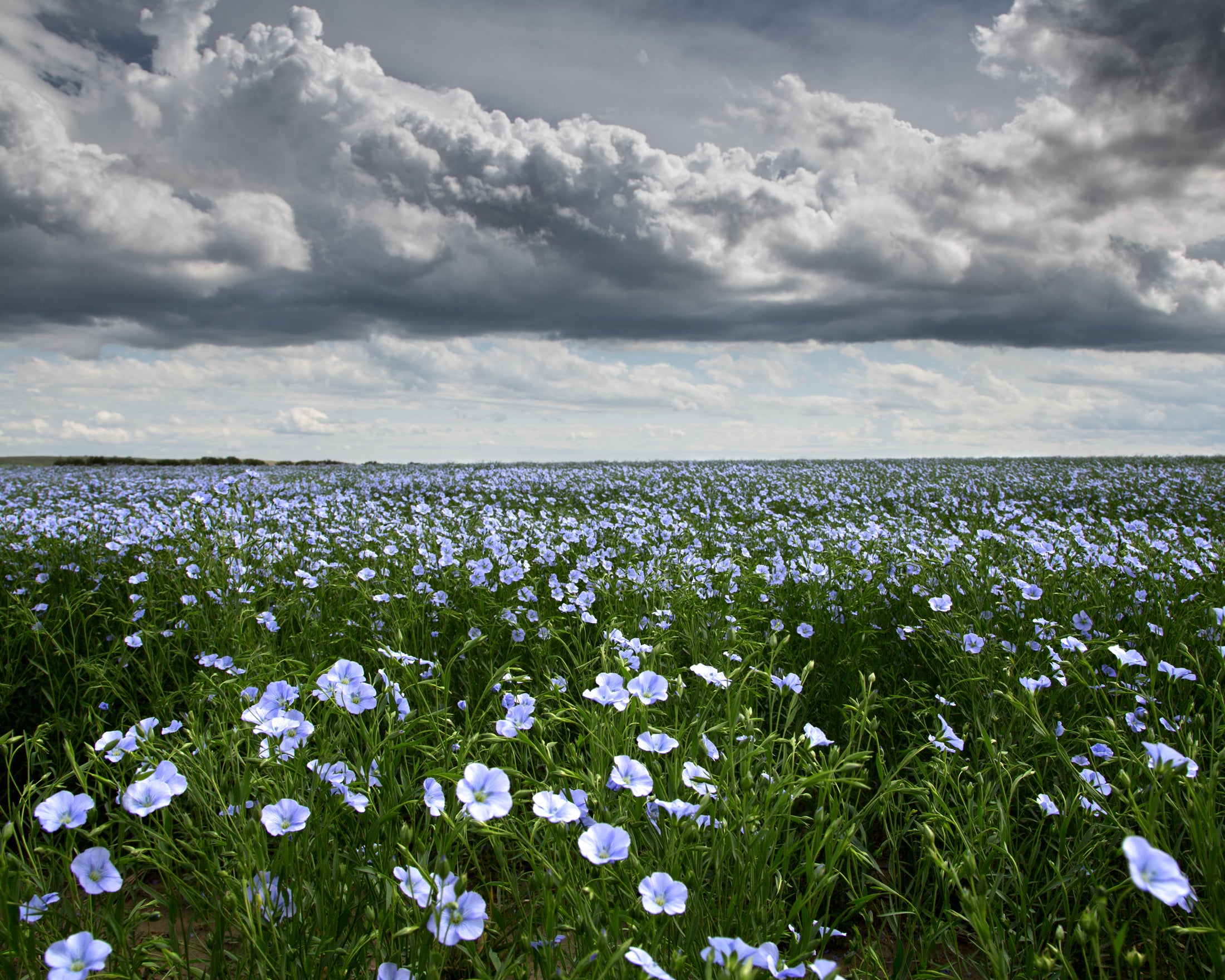The color photograph captures a vivid and enchanting field of light gray-blue flowers, likely resembling morning glories or flax flowers, spread across the lower half of the image. These trumpet-shaped blooms with five petals emerge from a sea of lush green grass, creating a dense and vibrant floral carpet. As the eye moves towards the horizon, the intensity of the flower concentration increases dramatically.

Above this blooming spectacle, the sky transitions into a dramatic scene filled with an array of cloud formations. The upper half of the image showcases thick, smoky gray clouds with lighter white patches interspersed, creating a stark contrast with the lower floral field. In the upper right corner, portions of the clouds turn darker, almost black, adding to the overall atmospheric tension. The interplay between the densely packed flowers below and the turbulent, heavy clouds above forms a compelling and dramatic visual narrative.